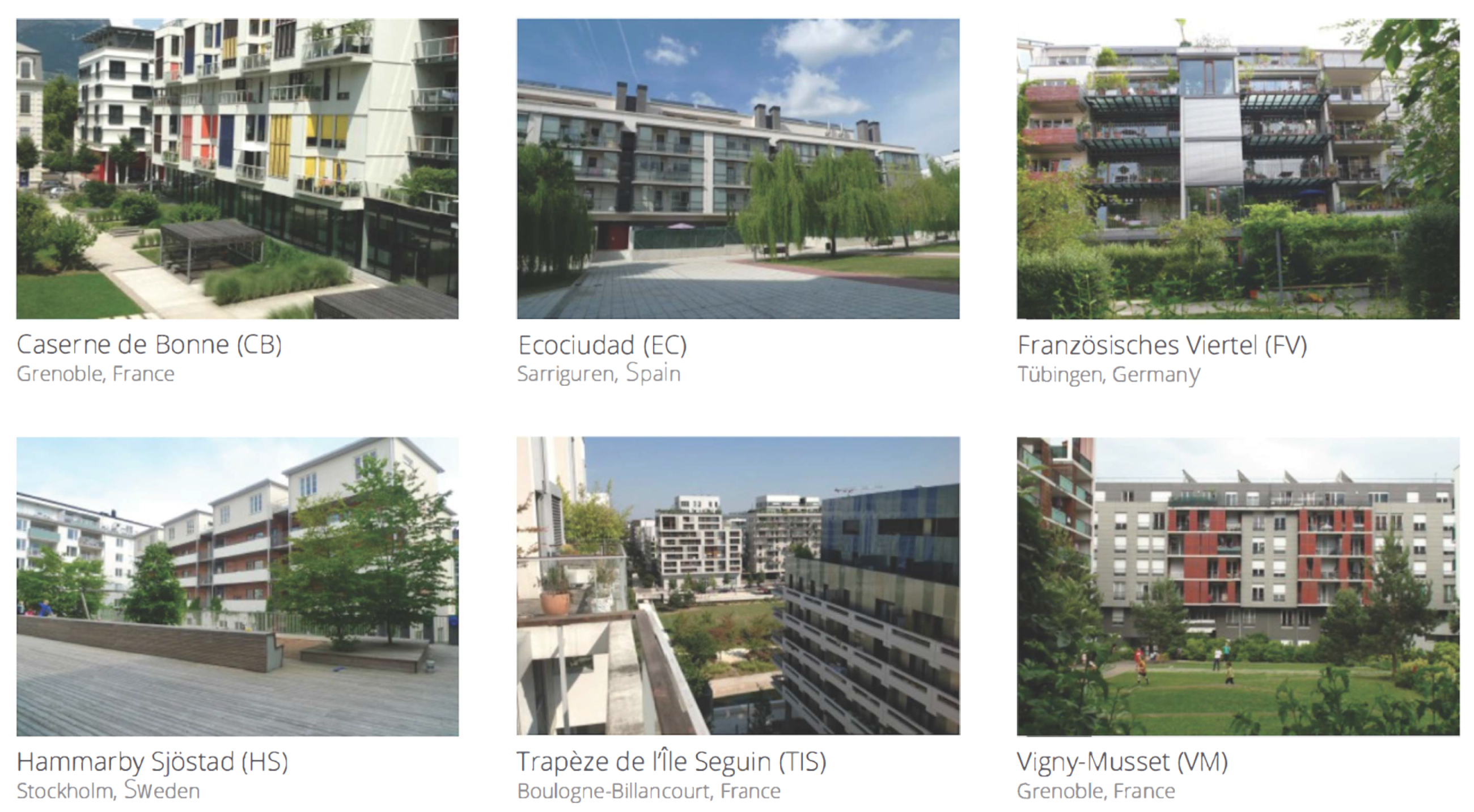This collage features six images showcasing various architectural landmarks from different European countries:

1. The Caserne de Bonne in Grenoble, France: A vibrant multi-colored building adorned with shades of yellow, blue, pink, and white. The front facade stands out with its eclectic palette, set against the backdrop of the picturesque city.
   
2. A prominent structure in Spain: This large brick building is surrounded by an array of lush trees, and it features a brick-paved driveway leading up to its grand entrance.
   
3. A notable edifice in Germany: This three or four-story building showcases balconies along its side, accentuated by meticulously maintained hedges, creating a refined and elegant appearance.
   
4. An imposing white building in Sweden: Nestled among numerous trees, this expansive structure exudes a sense of tranquility and grandeur.
   
5. A collection of large white buildings in another part of France: These substantial structures present a unified and impressive sight, standing tall and majestic.
   
6. A diverse array of buildings in France: Featuring a mix of red and gray hues, this cluster of long buildings displays a pleasing architectural variety, adding to the visual appeal of the scene.